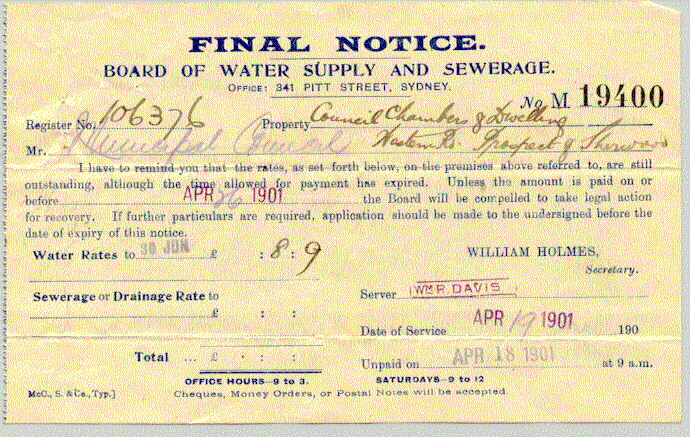This image captures an old, horizontally rectangular water company notice, printed on a yellowish cream background with black text and some blue bolded titles. The top of the notice prominently displays "FINAL NOTICE" in capital letters and underlined, followed by "Board of Water Supply and Sewerage," and the office address: "341 Pitt Street, Sydney." The document, marked with Number M19400 and Register 106376, is identified as the property of Council Chambers.

The text is partly handwritten and faded, making some parts difficult to decipher. It addresses a "Mr. [Indistinguishable Name]" in cursive, notifying them that the water and sewerage rates for the specified premises are still outstanding. Despite the payment deadline having passed, the required amount must be paid by April 26, 1901, to avoid legal action. The notice specifies further particulars can be sought from the undersigned before the expiration date of April 26, 1901.

Additional details include that the rates were last set on June 30, 1989, with William Holmes serving as Secretary. The server responsible is W. W. William R. Davis. The document also states the date of service as April 19, 1901, and notes the amount unpaid as of April 18, 1901. Payment options include checks, money orders, or postal notes, and the office hours are listed as 9 to 3 on weekdays and 9 to 12 on Saturdays. The bottom of the form reads MCC and something TIPP, further adding to its official nature.